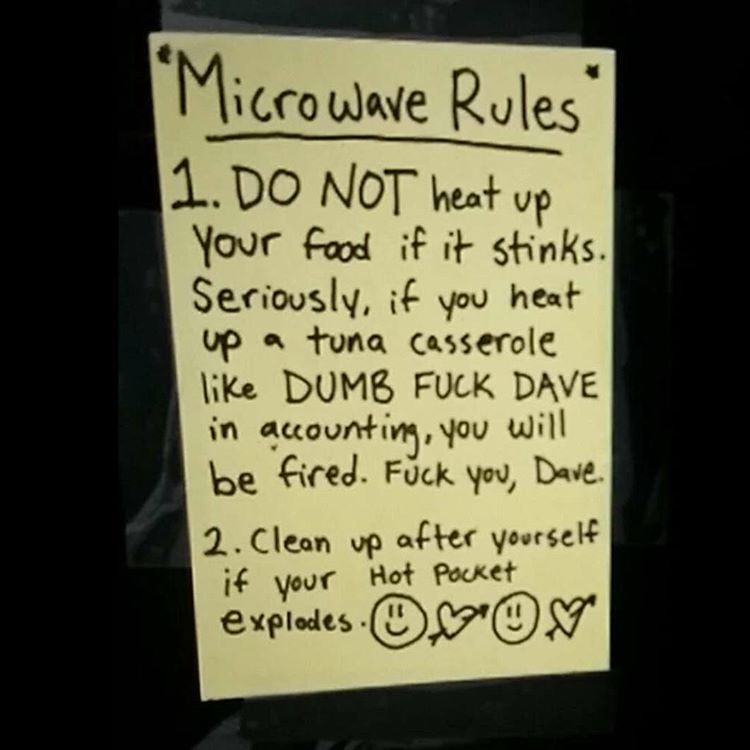The photo shows a cream-colored or off-white sheet of heavy paper, affixed slightly crookedly against a solid black background. Written in bold black marker, the sheet bears the title "Microwave Rules," with the title underlined and accompanied by decorative stars.

The rules are as follows:

1. "DO NOT heat up your food if it stinks. Seriously, if you heat up a tuna casserole like dumb fuck Dave in accounting, you will be fired. Fuck you, Dave."
2. "Clean up after yourself if your hot pocket explodes."

The message is embellished with two smiley faces, a heart with an arrow through it, and another heart towards the bottom-right corner, adding a sarcastic touch to its otherwise stern tone.